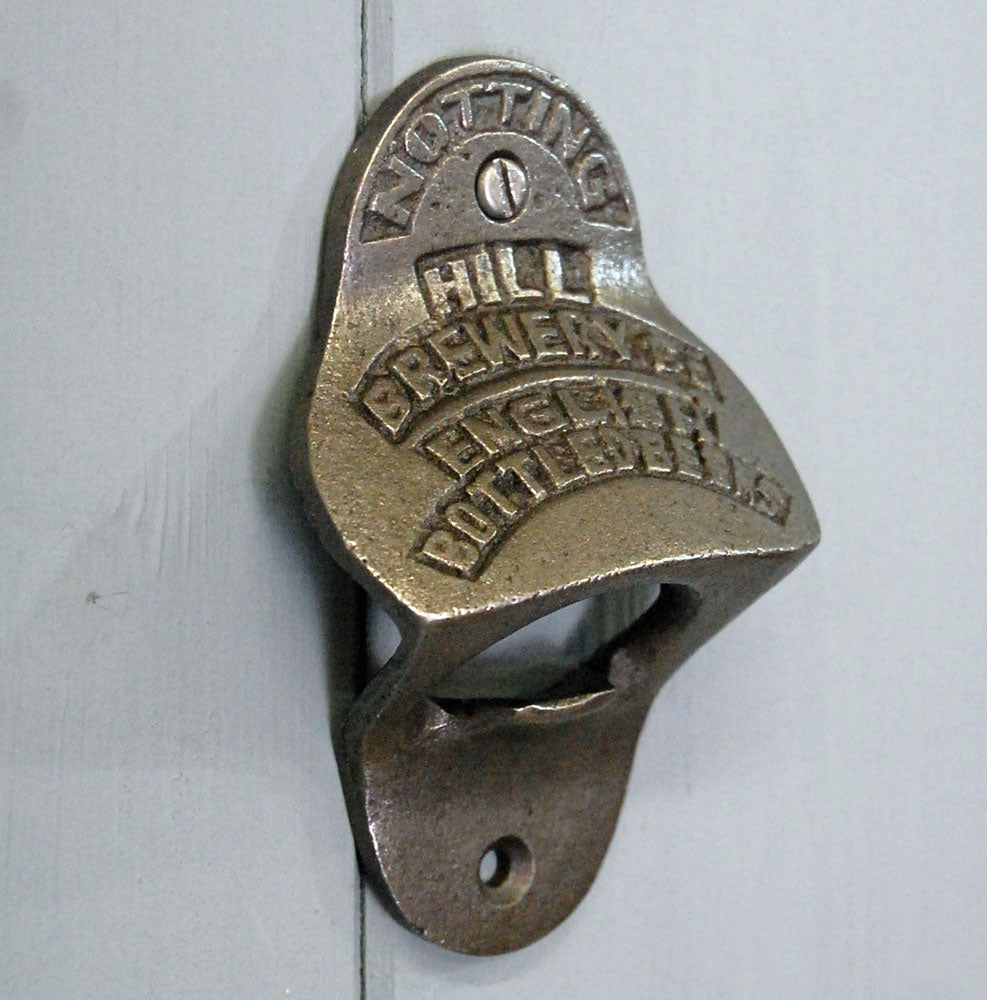This close-up photograph captures a metal bottle opener mounted on a wooden wall painted in a light, neutral color, possibly white or light gray. The bottle opener, made of a metal that has a brownish hue—almost a cross between gold and brown—features a slightly arced and angled design. It is secured to the wall with a single screw at the top, while the lower screw hole lacks a screw, indicating it could be more securely attached given its purpose. The embossed text "NOTTING HILL BREWERY ENGLISH BOTTLED BEERS" in sans serif, all capital letters, is clearly visible, though some letters are partially obscured due to the angle of the bottle opener. The text arcs along the rounded top and middle sections of the opener. Despite the missing bottom screw, the opener remains firmly in place on the wall, positioned slightly to the right, further enhancing its functionality and aesthetic appeal.